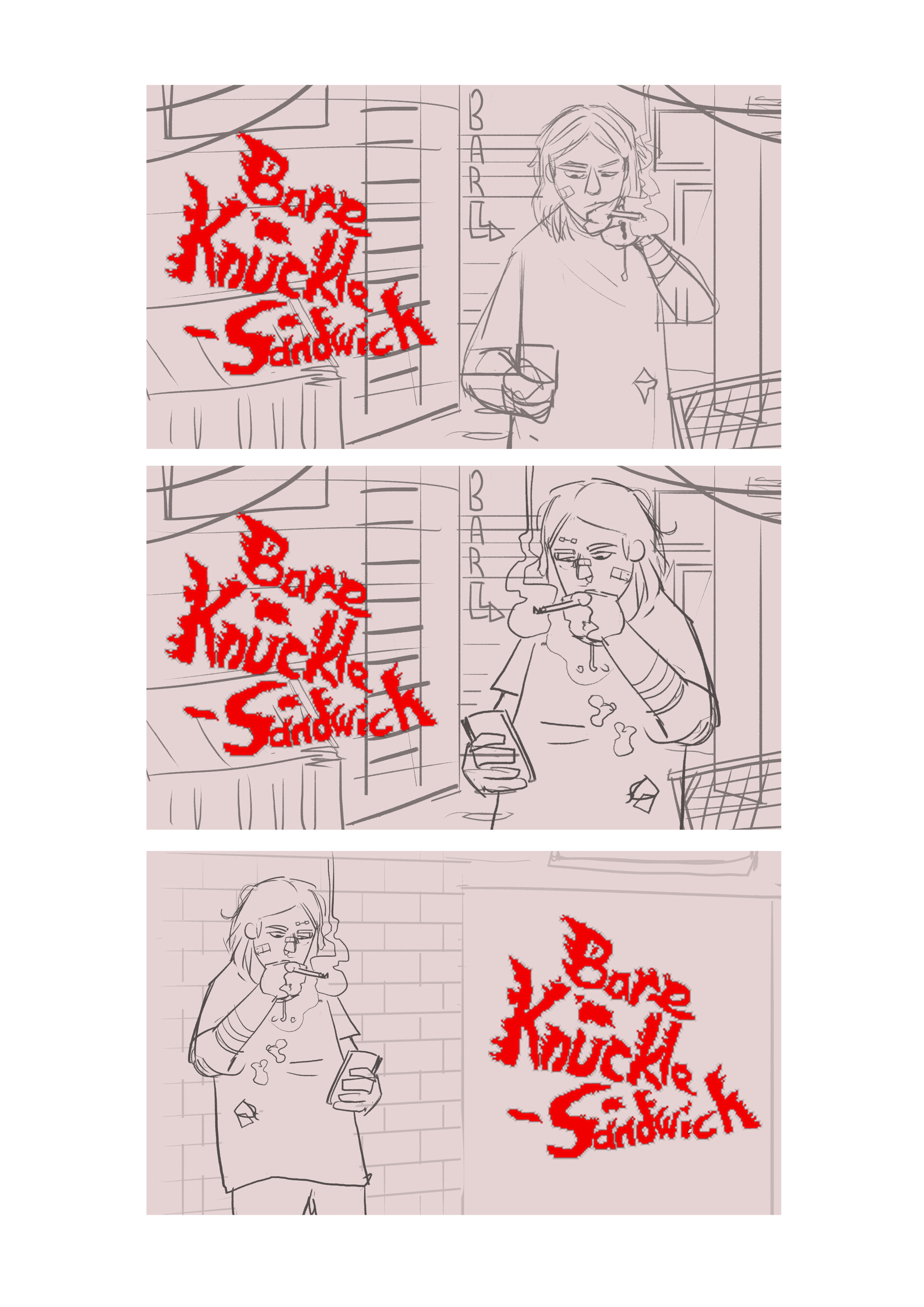The image is a series of three sketched drawings, presented vertically, each depicting the same person in a room, smoking a cigarette and looking at his phone. The artwork, done against pink backgrounds, portrays the figure from slightly varying angles. The character has long, scruffy hair, wears tattered clothing, and has bandages on his face, indicating a rough, possibly fighting-related lifestyle.

In the top two images, the setting includes a charcoal pencil sketch of the word "Bar" with an arrow pointing, suggesting a bar scene. The figure is consistently shown holding a cigarette and a phone, with the logo "Bare Knuckle Sandwich" prominently displayed in evocative red flame-esque lettering across each drawing. Details such as clothing stains and facial bandages become more apparent from the first to the second image, emphasizing a sense of increasing wear and tear.

In the last drawing, the composition shifts slightly: the "Bare Knuckle Sandwich" logo moves to the right of the figure, now leaning against a brick wall. The bar sign is no longer visible, focusing entirely on the individual who remains absorbed in his phone, cigarette in mouth, further solidifying the gritty, resilient nature of the character.